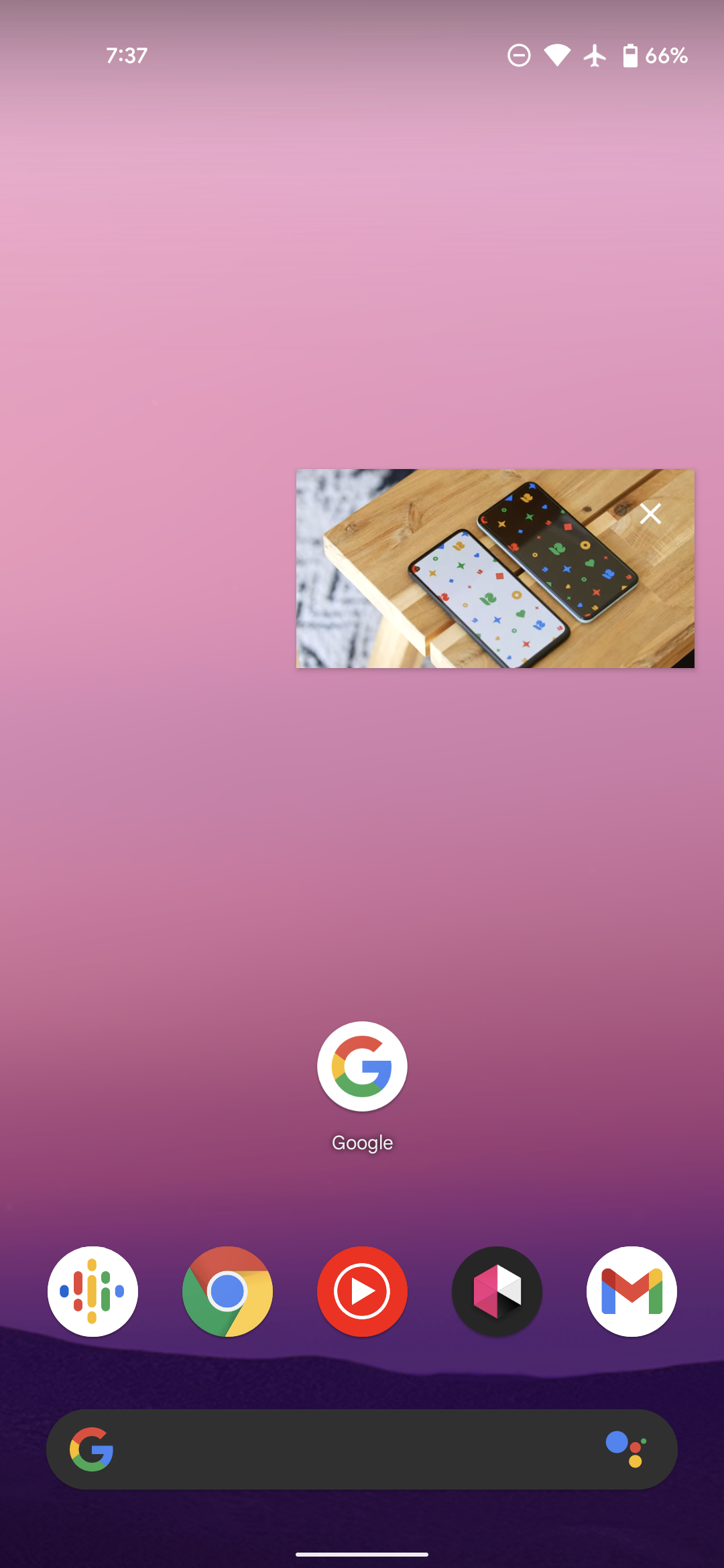This screenshot captures the home screen of a cell phone adorned with a gradient background. Starting from the bottom, a rich dark purple band transitions smoothly into a lighter purple hue before blending into a soft pink, culminating in a darker shade at the top. 

At the top-left corner, the time is prominently displayed in white as "7:37". The upper-right section features a series of icons: the "Do Not Disturb" symbol, a Wi-Fi icon, an airplane mode emblem, and a battery icon showing a 66% charge.

Anchoring the bottom of the screen is a Google search bar, easily identifiable by its colorful, capital "G" and assistant dots to the right. Just above, a row of application icons is lined up. From left to right, these include a Google product icon, the Google Chrome browser, either an Apple Music or YouTube app (defined by a red circle with a white play button in the center), an unidentified icon, and the Gmail app.

Centrally located above the application dock is a large Google widget alongside an image of two cell phones resting on a wooden bench. This organized yet visually appealing setup effectively highlights the user's app preferences and personalization.